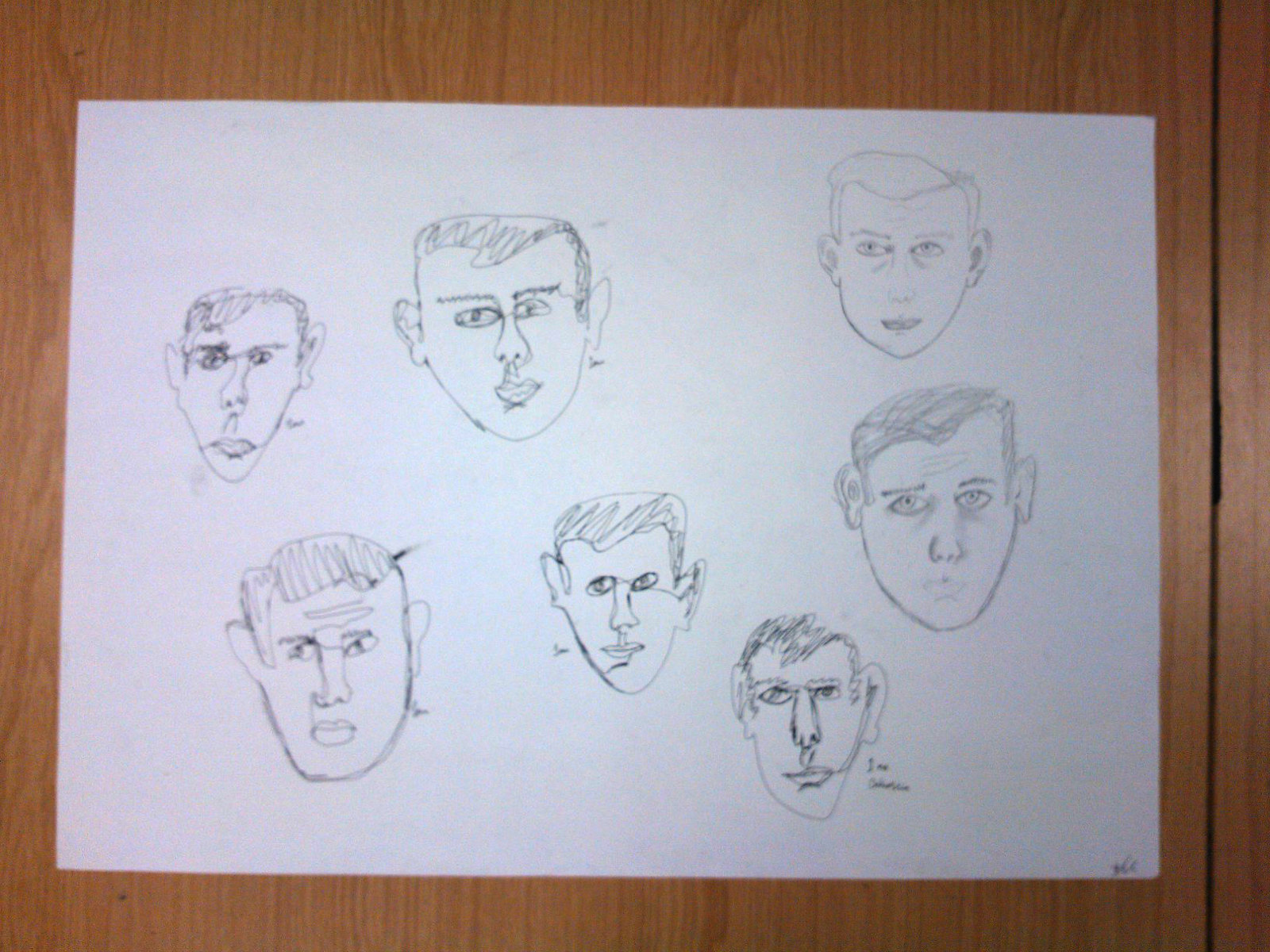The photograph captures a top-down view of a white piece of printer paper oriented horizontally (hamburger style) on a wooden desk with a plastic finish that has an orange wood swirl pattern. On the paper are seven simple line-art drawings of a man's head, each drawn in pencil and featuring slightly different art styles, suggesting multiple artists. The faces have basic shapes with almond eyes, thin noses, and simple mouths. Hair on each head is indicated with scribbled shading, and the eyes and noses have distinct but irregular shapes. The paper includes a small, illegible scribble in the lower-right corner that resembles a signature. The wooden desk underneath is a light brown with noticeable dark grooves.